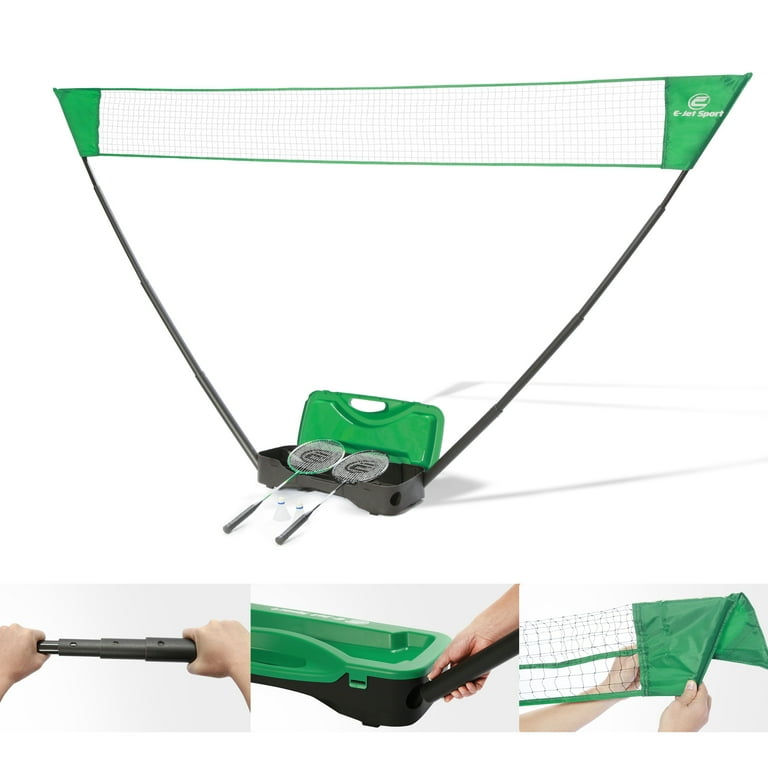The image depicts a portable badminton net system branded with "E-Jet Sports." The net setup comes in a compact, suitcase-like carry case. The case, which is primarily black with vibrant lime green accents matching the net, houses the entire setup, making it easy to store and transport. The system includes detailed assembly instructions at the bottom of the image, showing how to erect the net by extending black poles from the sides of the case and arranging them in a V-shape. The poles' tension ensures the net stays upright. Additionally, the package includes two rackets, one green and one black. Although the set does not explicitly show a shuttlecock, it implies sufficient space within the case for all necessary game equipment, making it a complete kit for a portable badminton match.